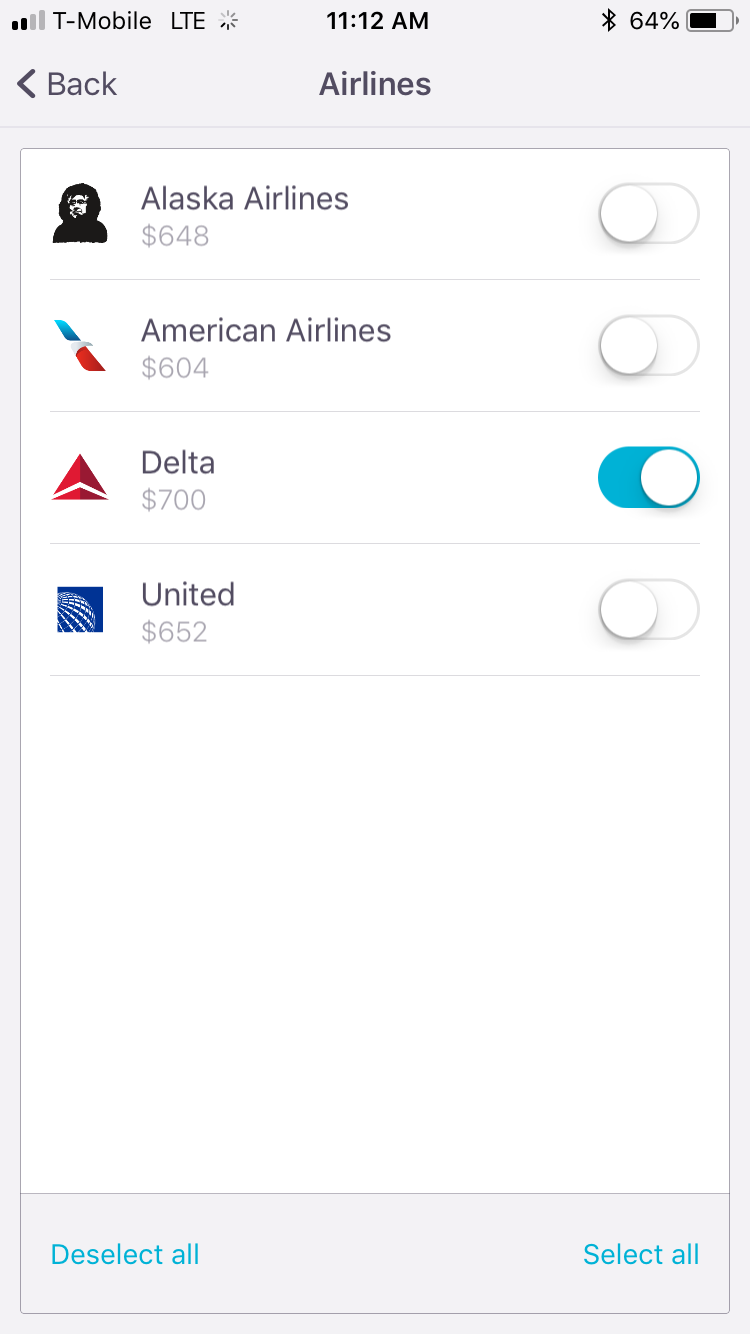Certainly! Here's a detailed and cleaned-up caption:

"In this smartphone screenshot, we see a grey background. In the top-left corner, there's a status bar with a signal strength icon partially colored in black and grey, indicating 'T-Mobile LTE' with a buffering signal. To its right, the time is displayed as '11:12 AM' and further right, the battery icon shows '64%' life remaining.

Directly below the status bar, on the left, there's a black arrow pointing left with the word 'Back' beside it. In the middle header section, it says 'Airlines' above a thin grey line.

The content section is framed by a grey outline. The first entry features a black and white image of a person, labeled 'Alaska Airlines' with a secondary text in lighter font that says '648', and a white circle indicating it is not selected.

The next entry below has a logo with blue and red colors and a bird's face, labeled 'American Airlines' in black font. The secondary text in grey says '604', also with a white circle indicating it is not selected.

The third entry, separated by another grey line, shows a red triangle logo split by a break line, labeled 'Delta' in black font. The secondary text in grey says '$700'. This entry features a blue dot in a powder blue circle, indicating it is selected.

The final item in the list shows a blue box with white lines in a circle, labeled 'United' in black font. The secondary text says '652', and the white circle indicates it is not selected.

At the bottom, there is a grey box with blue text on the left saying 'Deselect All' and on the right saying 'Select All'. A grey line runs underneath this section, merging with the grey background that extends from the top to the bottom of the image."

Feel free to let me know if you need anything else!